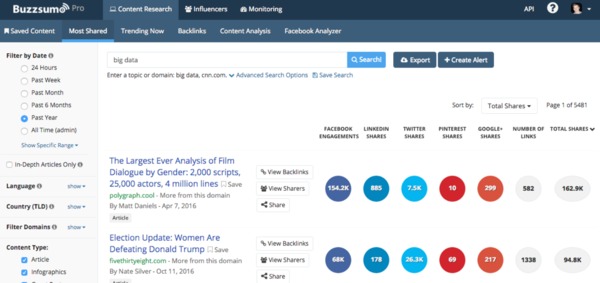Here is a cleaned-up and detailed caption:

---

This screenshot from BuzzSumo Pro features the site’s user interface. The "BuzzSumo" logo is prominently displayed in white font, while "Pro" is in gray, set against a black background. Beside the logo are key sections for navigation: Content Research, Influencers, and Monitoring. Below these primary sections are additional clickable options: Saved Content, Most Shared, Trending Now, Backlinks, Content Analysis, and Facebook Analyzer.

In the main view, the user has selected the "Most Shared" content filter, set to display data from the "Past Year." The timeframe filter offers a range of options from the past 24 hours to all-time. Below these filters, options are provided for specifying languages, countries, domains, and content types such as articles or infographics.

To the right, the interface displays a list of highlighted stories. The top story is titled "The Largest Ever Analysis of Film Dialogue by Gender," covering 2,000 scripts, 25,000 actors, and 4 million lines. Following that, there is an article titled "Election Update: Women Are Defeating Donald Trump." Adjacent to the stories are social media engagement metrics, including interactions from platforms like Facebook, LinkedIn, Twitter, Pinterest, Google, and more.